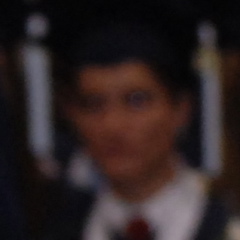This is a small, color photograph featuring a man captured from the chest up. He appears to be dressed in a formal suit, with a white shirt and a red tie. The man's hair is short, and he is looking slightly to one side. The image quality is notably poor, making his facial features indistinguishable, though the dark areas of his eyes are barely visible. In the background, there are two white poles positioned on either side of the frame, one on the left and one on the right.